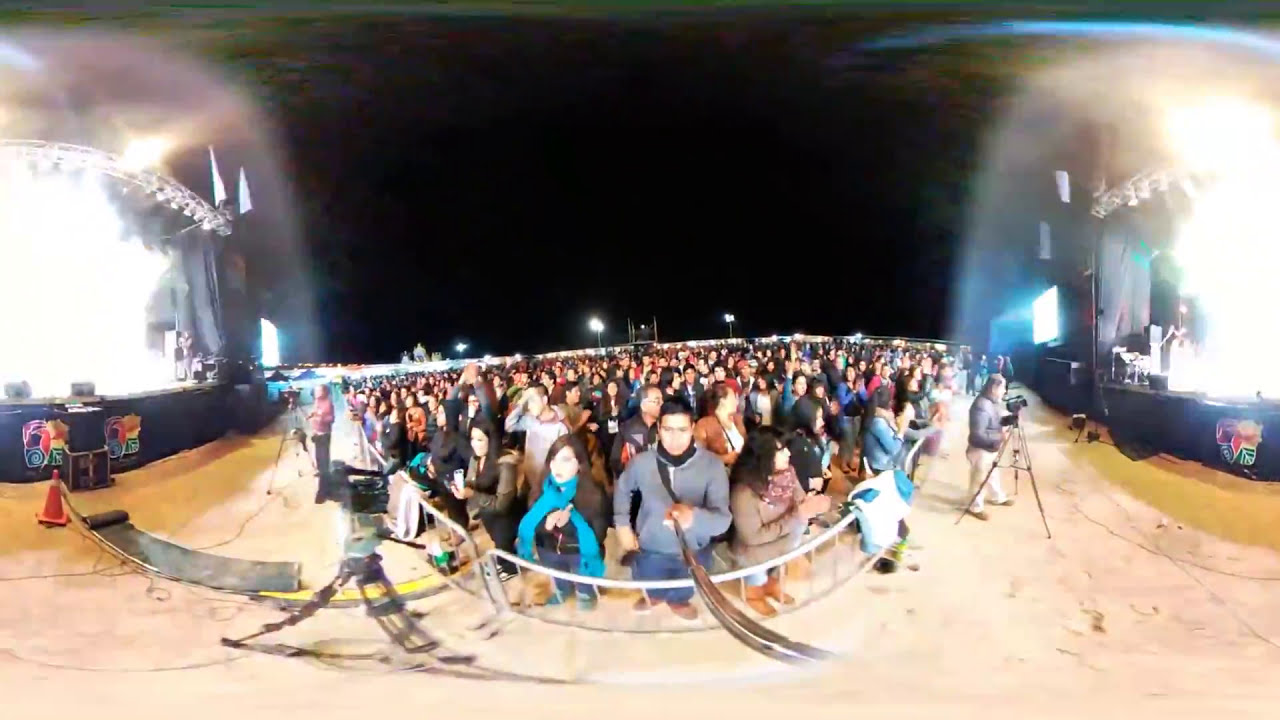The image captures a vibrant nighttime scene at a music festival, taken with a fisheye or panoramic lens, giving it a wide-angle perspective. The scene is dominated by a vast crowd of people, densely packed and centered in the image, indicating a high-energy environment. They appear to be dressed for cool weather, many wearing coats and jackets. The foreground features a sandy surface, and the background is marked by a dark sky suggesting nightfall. 

On either side of the image, stages are visible, both brightly lit and featuring barricades that keep the crowd at bay. A noticeable detail includes a man at the center using a very long selfie stick to capture a picture, dressed in a gray hoodie, black undershirt, jeans, and brown shoes. Flanking him on each side are two young women. Additionally, another cameraman with a tripod is set up near the stage on the right side of the image. The color palette is diverse, with shades of black, light blue, yellow, red, purple, green, gray, and white scattered throughout. The entire scene is framed by the dark, expansive nighttime sky, encapsulating the buzzing atmosphere of the outdoor concert.